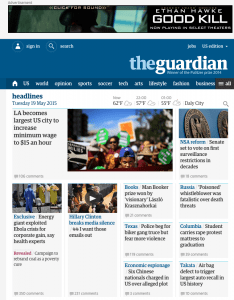This screenshot captures a user's tablet displaying a webpage from The Guardian, a prominent news information site. At the very top of the screen, there is an advertisement featuring the movie "Good Kill," starring Ethan Hawke, though the image is dark and somewhat difficult to discern. Beneath the ad, the main headline stands out in large font, announcing that Los Angeles has become the largest U.S. city to raise the minimum wage to $25 an hour. Although the other headlines are blurry, the page includes three additional photographs, making a total of four images on the screen. The Guardian’s website features a medium shade of blue prominently across the top of the homepage, adding to the overall layout's visual coherence.